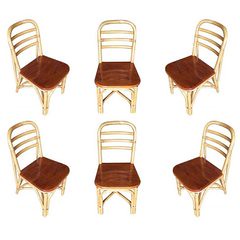This detailed photo showcases six miniature chairs arranged in two rows of three. The middle chairs in both rows are facing directly towards the camera, while the outer chairs are angled inwards, pointing towards the central chair in each row. Each chair features a shiny, coppery or faux wooden rounded seat and a golden metal frame, including four golden legs. The backrest consists of a golden arch with three horizontal bars beneath it, creating a partially open back. Additionally, there is an internal cross-bracing under the seat, forming an X-shape for added support. The meticulous design of these chairs adds a unique and elegant touch to the arrangement.